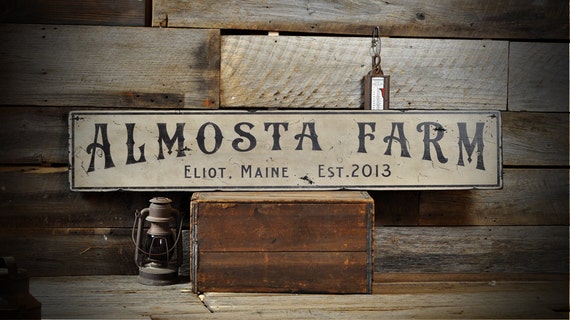This is a close-up image of a white, wooden sign with black lettering, reading "Almost a Farm, Eliot, Maine, Established 2013." The sign is positioned inside what appears to be a wooden building, likely a barn, and is resting on a block of wood. To one side of the block, an oil lamp is situated beneath the sign. On top of the sign, there's another type of lamp with a silver base. The floor, made of wood, unmistakably suggests the rustic ambience of an old barn.